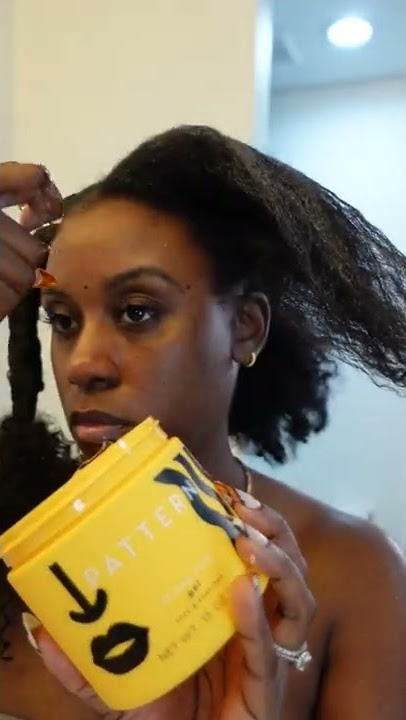In this photograph, a young black woman, estimated to be between 25 to 40 years old, is seated in a beauty salon, engaged in a hair braiding session. Behind her is a white wall to the left and a bluish-tinted wall to the right, featuring recessed lighting in the ceiling. The focal point of the image is the elaborate braiding process in her hair, which shows considerable progress. She appears slightly bored, gazing off into the distance and not making eye contact with the camera.

The woman is elegantly adorned with a small hoop earring in her left ear, which appears either gold or silver, and she wears a sizable diamond engagement ring on her left hand's ring finger. Her fingernails are notably long, well-manicured, and painted a light color. She holds a vibrant yellow jar labeled "Pattern," prominently displaying black lips and arrows pointing down, most likely a hair product for her beautician to use during the braiding. Additionally, a pair of visible black hands with an orange tool can be seen at her forehead, assisting in the hair treatment. The detailed and stylish touches, such as her potential necklace and immaculate nail care, underscore her attractiveness and attention to personal grooming.